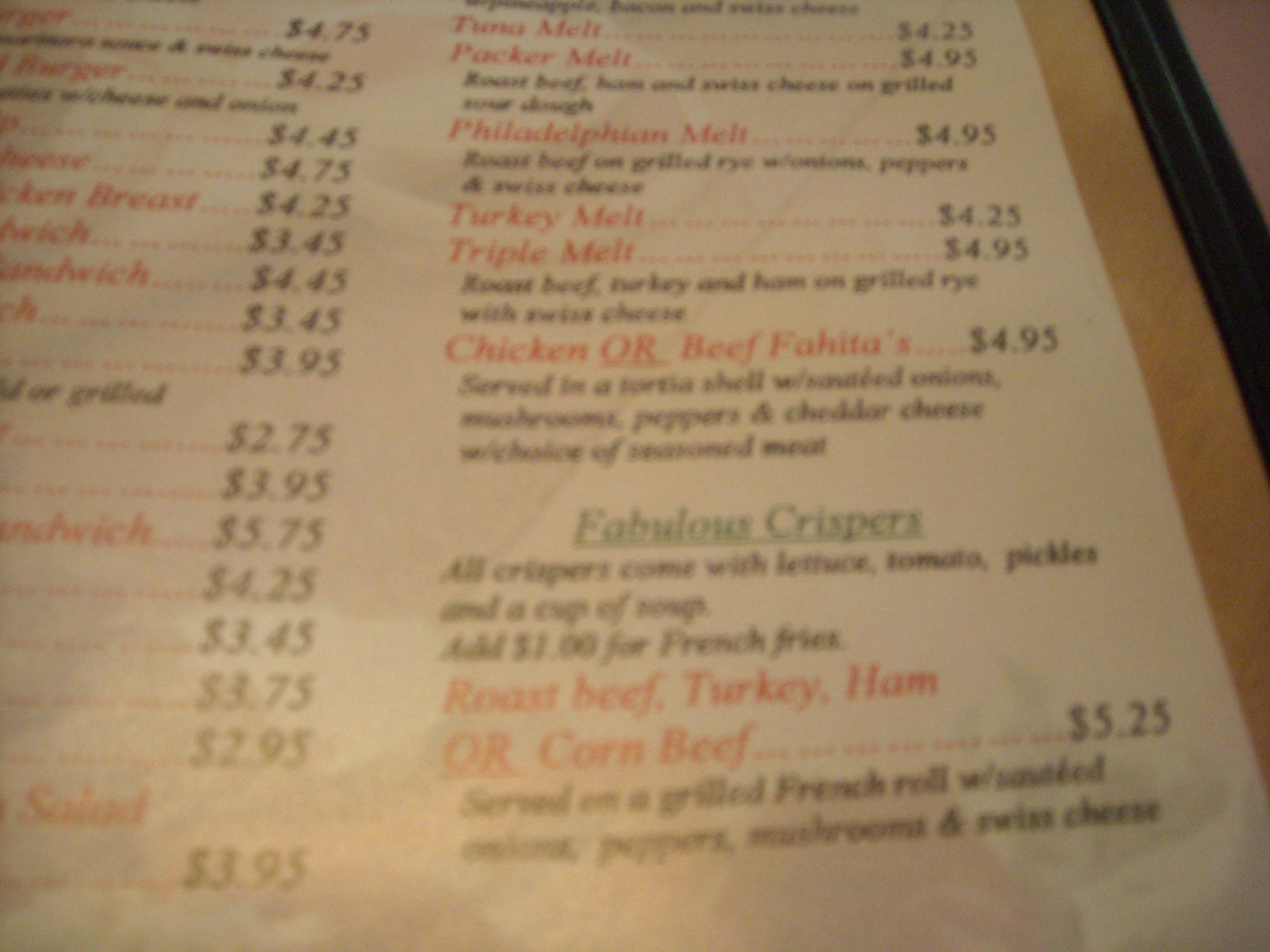A close-up, landscape-oriented image captures a slightly blurry and out-of-focus restaurant menu. The menu itself rests on a table with a light tan wooden surface bordered by black trim, possibly part of the table. The menu's design includes a white background with a mix of red and black text. Key items are listed in red, such as "Tuna Melt" with a price of "$4.25" in black text. Similarly, "Packer Melt" is listed with a price of "$4.95" in black. Further menu items include "Philadelphia Melt," "Turkey Melt," "Triple Melt," and "Chicken or Beef Fajitas," each accompanied by descriptions in black text below the item name. The next section of the menu is introduced with the phrase "Fabulous Crispers" in green letters, indicating a shift to a different category of offerings.